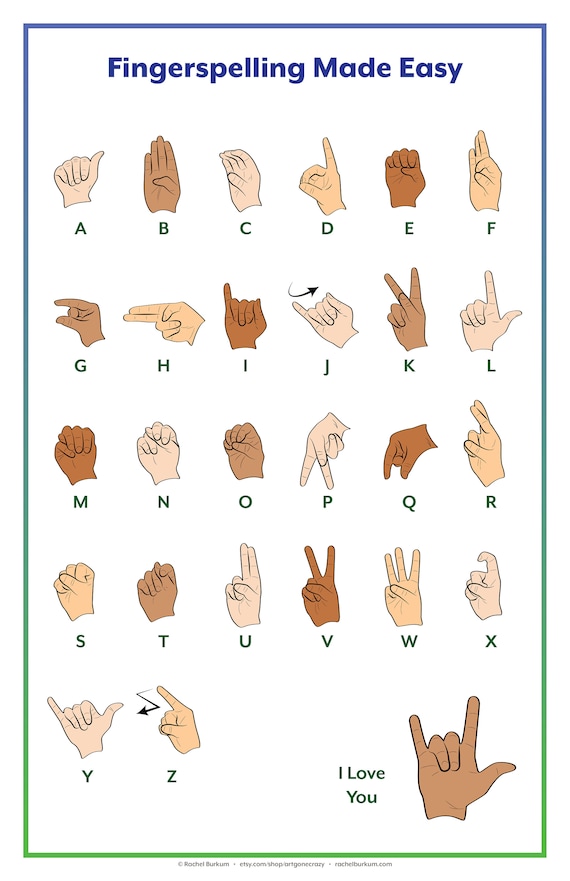This cartoon or synthesized image illustrates a comprehensive chart of the American Sign Language (ASL) alphabet. The background is crisp white, and a long rectangular border encapsulates the chart. The border displays a gradient that fades from blue at the top to bright green at the bottom. At the top of the chart, prominently written in dark blue, is the title "Finger Spelling Made Easy."

The chart itself is divided into columns and rows: five rows of six columns display vector-drawn hands, which are stylized to represent different skin tones—ranging from light peach to darker browns and middling hues—depicting each letter of the ASL alphabet. Each hand sign aligns with a letter, written underneath in green. The rows present the letters A through Z in this sequential arrangement:

1. A, B, C, D, E, F
2. G, H, I, J, K, L
3. M, N, O, P, Q, R
4. S, T, U, V, W, X
5. Y, Z (the fifth row is shorter, only two-columns wide)

In the bottom right-hand corner, a hand is positioned in the "rock and roll" symbol, doubling as the ASL sign for "I love you," with the index finger, little finger, and thumb extended. Beside this hand, "I love you" is written in green. Below the chart's border, there is a small line of black text, although it is too minuscule to be legible.